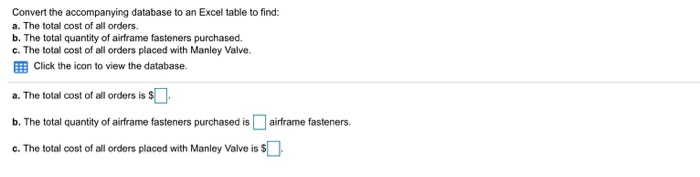This image on a white background contains black text organized into two main sections, separated by a horizontal gray line.

**Top Section:**

- **Heading:** "Convert the accompanying database to an Excel table to find:"
- **Bullet Points (Bolded):**
  - **A:** The total cost of all orders.
  - **B:** The total quantity of airframe fasteners purchased.
  - **C:** The total cost of all orders placed with Manly Valve.

Underneath these points, there's a blue calendar icon with the text "Click the icon to view the database."

**Bottom Section:**

- Bolded bullet points with larger spacing:
  - **A:** "The total cost of all orders is $[green rectangle]."
  - **B:** "The total quantity of airframe fasteners purchased is [green rectangle] airframe fasteners."
  - **C:** "The total cost of all orders placed with Manly Valve is $[green rectangle]."

The formatted and detailed sections help guide the viewer on the tasks related to converting a database into an Excel table and further analyzing the presented data on purchases and costs.